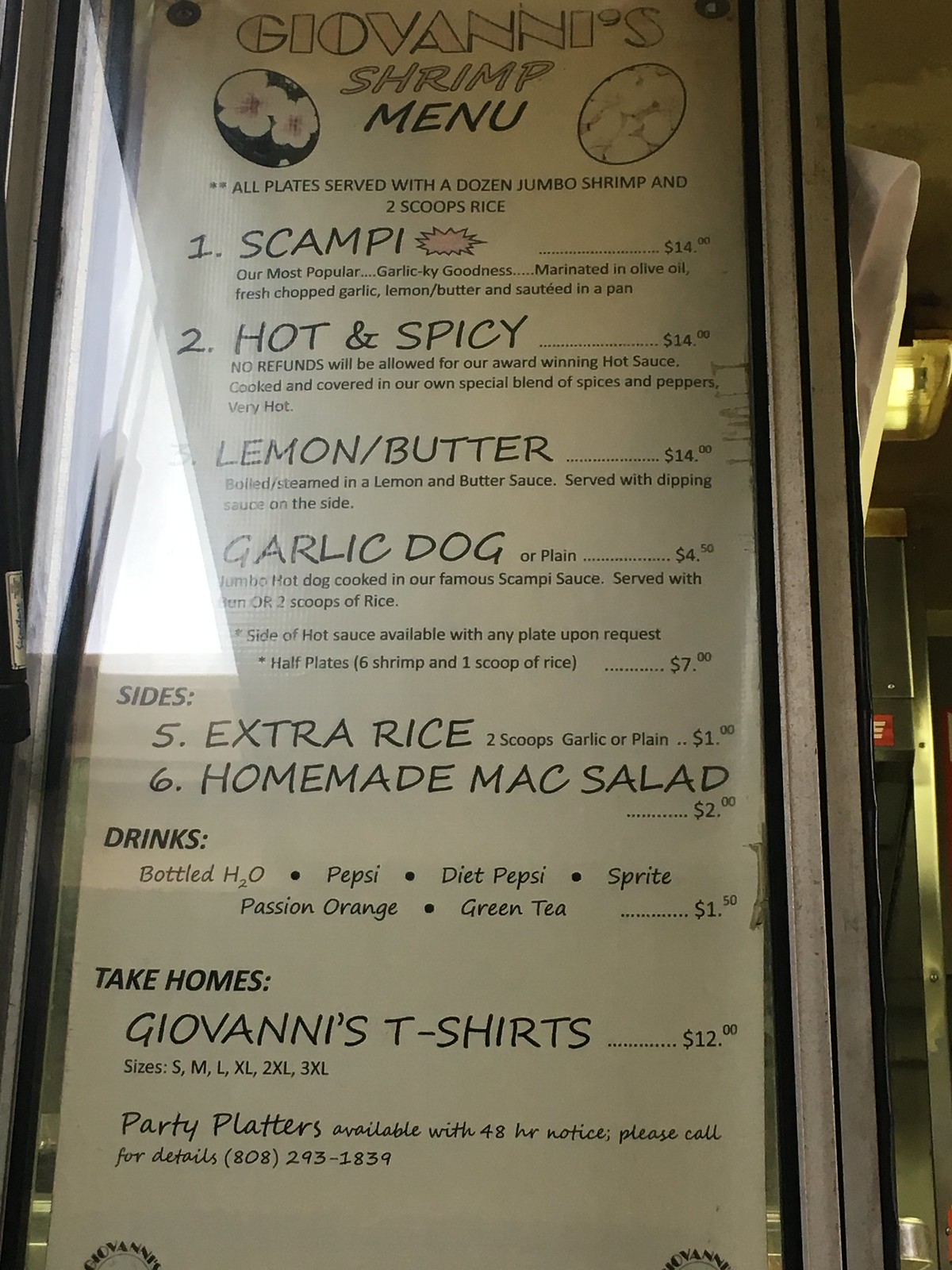This is a detailed color photograph of a menu displayed behind a glass panel. The upper left corner of the glass has a large reflection, slightly obscuring some of the text. The menu belongs to "Giovanni's Shrimp" and is prominently titled with the name "Giovanni's" spelled out clearly. 

To the left of the title, there is a circle featuring a photograph of two white flowers. On the right, another circle contains an unidentified illustration. The main menu text reads: "All plates served with a dozen jumbo shrimp and two scoops of rice."

1. **Scampi - $14**: This is described as the most popular dish, featuring garlicky goodness. The shrimp are marinated in olive oil, fresh chopped garlic, lemon butter, and sautéed in a pan. 
2. **Hot and Spicy - $14**: This dish, cooked in an award-winning hot sauce, is noted for being extremely hot and includes a special blend of spices and peppers. The menu warns that no refunds are available for this dish due to its heat level.
3. **Lemon Butter - $14**: Shrimp boiled or steamed in a lemon and butter sauce, served with a side dipping sauce.
4. **Garlic Dog or Plain - $4.50**: A jumbo hot dog cooked in Giovanni's famous scampi sauce. The detailed description is partially obscured by the reflection, but it also mentions an option for two scoops of rice.

The menu also notes that a side of hot sauce is available upon request. 

**Half Plates** offer six shrimp and one scoop of rice for $7. Additional **Sides** include:

5. Extra rice (two scoops, either garlic or plain) - $1
6. Homemade mac salad - $2

**Drinks** available are bottled water, Pepsi, Diet Pepsi, Sprite, Passion Orange, and Green Tea, each priced at $1.50.

**Take-home Items** include Giovanni's T-shirts for $12 in sizes ranging from small to 3XL. Party platters are also available with 48-hour notice, and the menu provides a contact number for details: 808-293-1839.